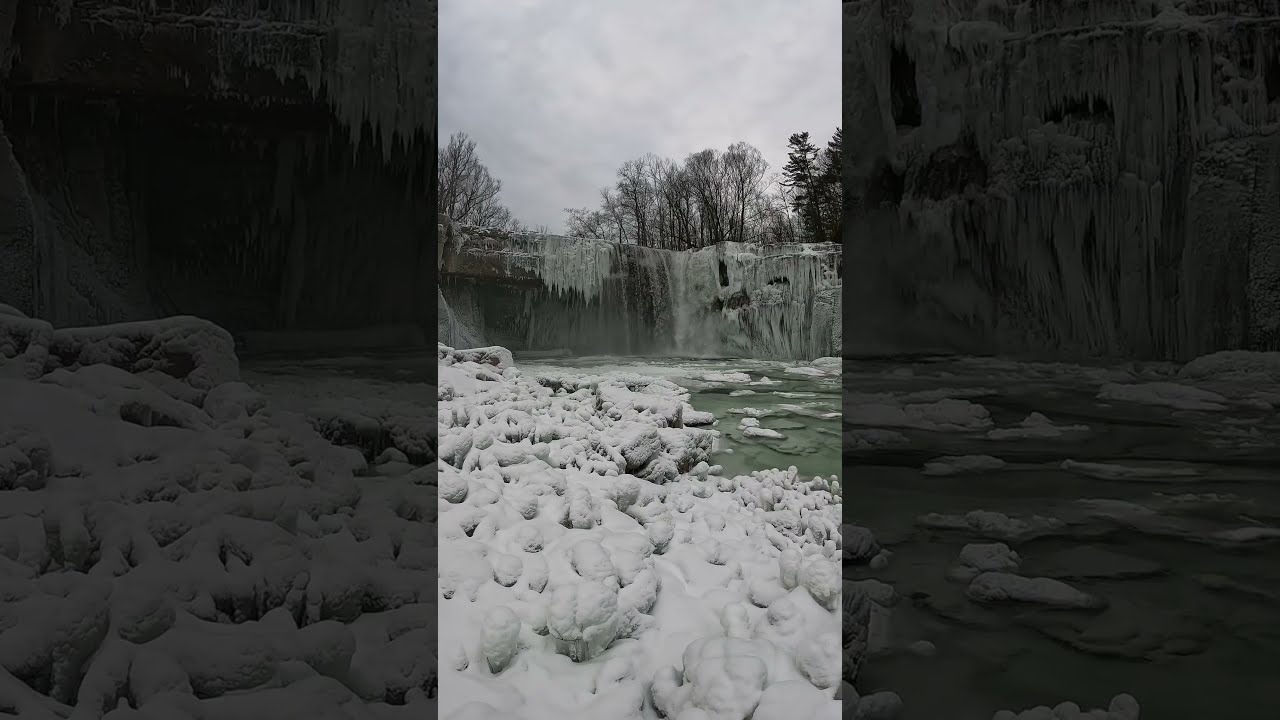The photo depicts an enchanting wintry scene, appearing on a cell phone screen. In the foreground, snow-covered mounds, possibly rocks, line the icy banks of a river or lake. The body of water itself hosts floating pieces of ice, with the unfrozen patches reflecting the stark, gray sky above, suggesting an imminent storm. In the background, a frozen waterfall drapes over a bridge or rocky ledge, creating an intricate display of icicles. Beyond this icy cascade, a serene winter forest with barren, leafless trees stands against the somber sky. The image is split into three panels, with close-ups on the left and right sides. The borders are composed of enlarged, slightly grayed-out segments of the main image, framing the central view and adding depth to the overall composition.